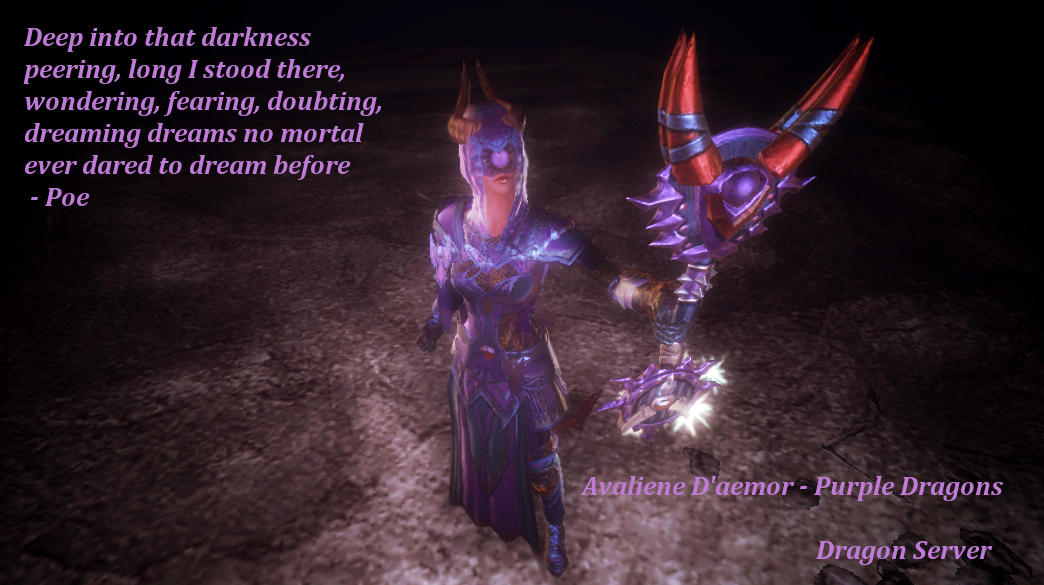The image is a screen capture from a video game, featuring a female warrior in a detailed, metallic-looking purple outfit. She is holding a large, intricate trident-like weapon that is purple with red horns and blue stripes, and it shines with a red glow at the bottom. The warrior wears a purple mask adorned with brown horns, obscuring her face. The perspective of the image is slightly elevated, looking down at her, standing on a gray, stone-like floor that has a patchy, dirt-like appearance. The edges of the image are dark, enhancing the focus on the illuminated central figure and her glowing weapon. In the top left corner of the screen, there is a quote: "Deep into that darkness peering, long I stood there, wondering, fearing, doubting, dreaming dreams no mortal ever dared to dream before. - Poe." The bottom right corner includes text in purple: "Ava Tiene de Amor, Purple Dragons, Dragon Server."